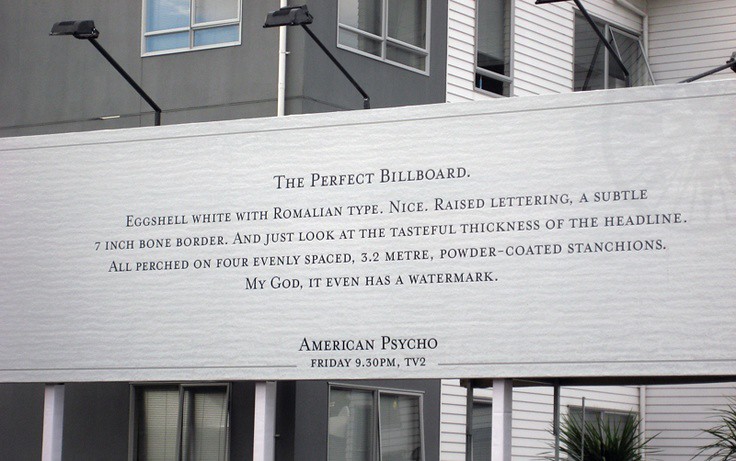This black-and-white photograph depicts a distinctive billboard, set against a backdrop of gray and white apartment-style houses. The rectangular billboard is supported by three square white posts and illuminated by three metallic arms with spotlights hanging over its top edge. The black text on the billboard reads, "The perfect billboard. Eggshell white with Romalian type. Nice, raised lettering. A subtle seven-inch bone border. And just look at the tasteful thickness of the headline. All perched on four evenly spaced 3.2 meter powder-coated stanchions. My God, it even has a watermark." This description humorously mimics the iconic business card scene from "American Psycho," and the billboard's bottom text attributes it to "American Psycho, Friday, 9.30 p.m., TV2." A faded compass watermark is visible in the upper right corner of the billboard, enhancing its detailed design.